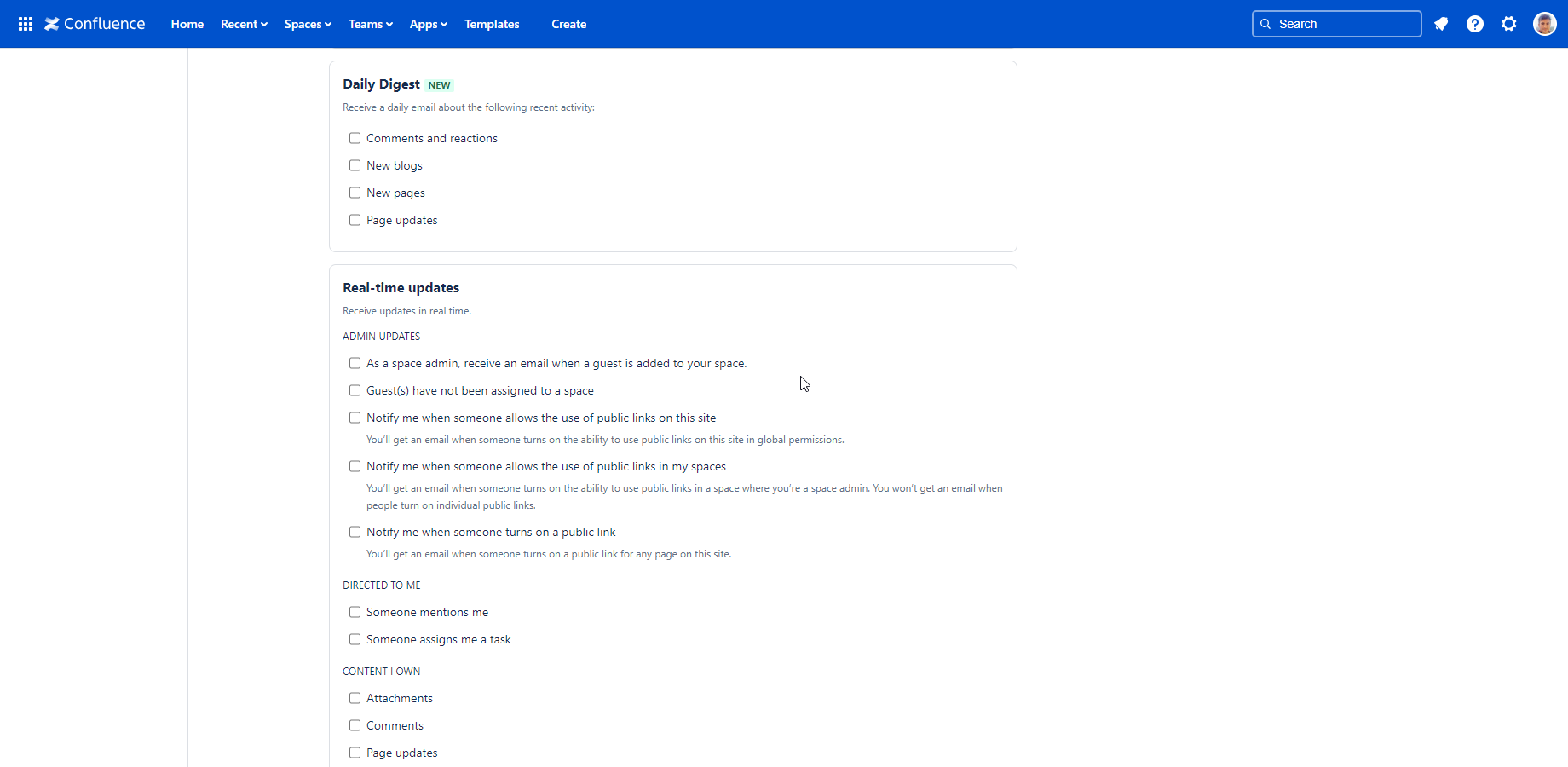This image is a detailed screenshot of a Confluence webpage with a white background. At the top of the page, there's a prominent blue bar with various elements. On the far left of the blue bar, there are two icons in white: the first icon is a 3x3 grid of dots, and next to it is a white 'X'. Following these icons is the text 'Confluence', indicating the name of the website. To the right of the site name, there's a clickable sitemap with links labeled "Home," "Record," "Spaces," "Tears," "Ages," "Templates," and "Create"—though some of these labels might be misinterpreted due to the small size of the screenshot. 

Continuing to the right, there is a search field indicated by a magnifying glass icon, followed by three more icons: a bell for notifications, a white circle with a blue question mark for help, and a gear for settings.

Below the blue bar, the main section of the webpage appears on a white background. The heading "Daily Digest" is in black font, followed by a line that is unreadable. Beneath this, there are several interactive checkboxes, each labeled with options: "Comment and Reaction," "New Blogs," "New Pages," and "Page Updates."

Overall, the screenshot captures a fragment of the Confluence interface with a focus on navigation menus and content settings.